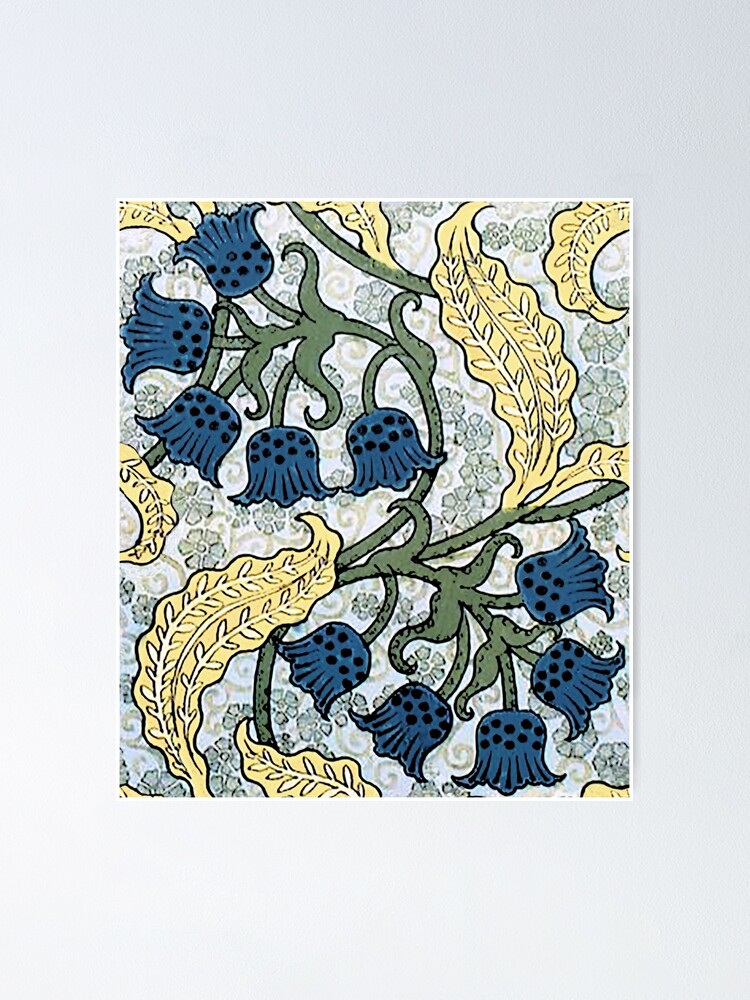This photo depicts a square art print set against a light gray background, framed with a thin white border. The painting features a vertical, organic floral design with olive green stems that curve elegantly from the bottom left to the upper left and then downward to the bottom right. Adorning these stems are multiple blue bell-shaped flowers dotted with black at their bases, totaling about eight to ten in number. Interspersed among the flowers are yellow leaves with visible veins, around five in count, adding to the intricate detailing. Additionally, there are softer, pale green blooms scattered in the background, seemingly not connected to the main stems. The entire artwork, rendered in either paint or colored pencil, evokes a sense of a classic, repeating wallpaper pattern, enhancing its decorative appeal.